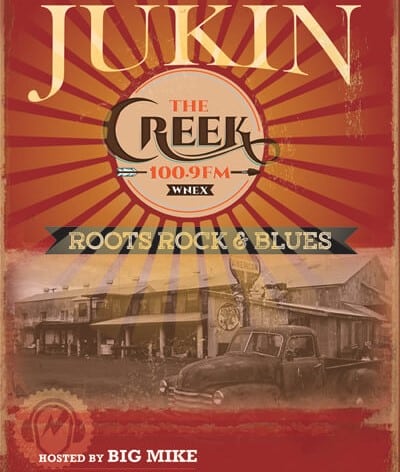The image is a small, vintage-inspired promotional poster dominated by red hues. At the top, bold yellow text announces "Junkin," beneath which a circular emblem with a sunray design prominently displays "The Creek, 100.9 FM, WNEX," with an arrow piercing through the "100.9 FM." Below this, a banner reads "Roots, Rock and Blues" in black lettering. The bottom half of the poster showcases a black and white photograph of a nostalgic scene featuring a mid-20th century Chevrolet pickup truck parked in front of an old gas station, with vintage storefronts and a higher warehouse-style building in the background. The lower left corner features a striking logo depicting a lightning bolt over a profile of a head with a microphone and headphones. The poster concludes with the text "Hosted by Big Mike" in yellow against a red backdrop.